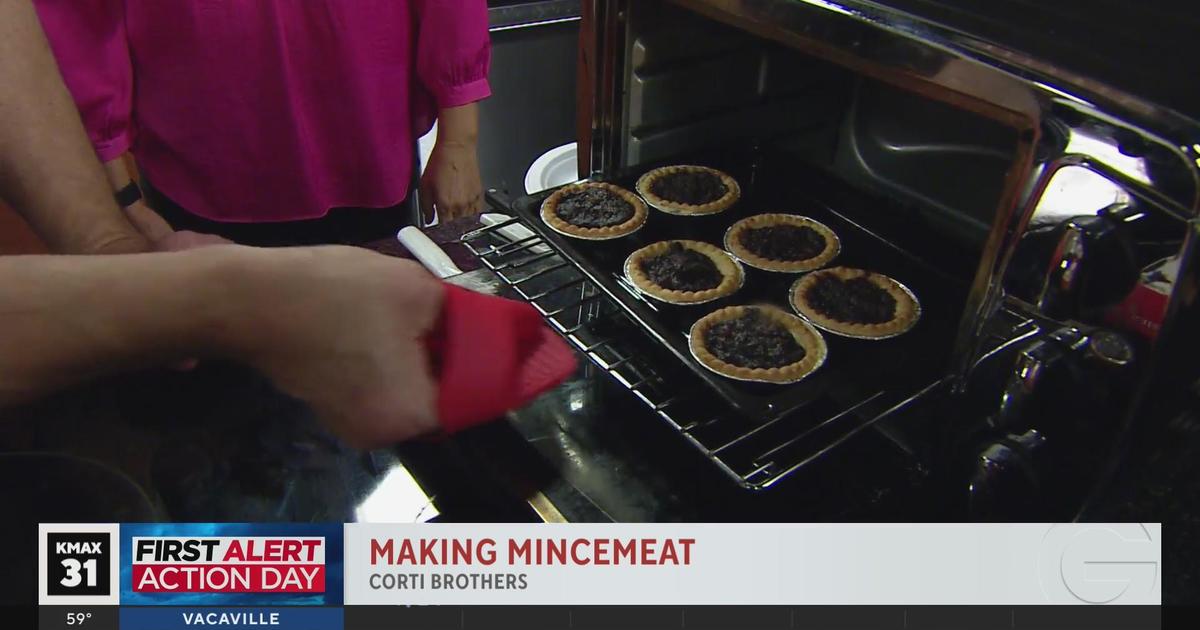The image captures a close-up scene of someone using a red oven mitt to pull a tray out of a toaster oven, with their hands and arms extending from the left side of the frame. The tray holds six small pies or tarts, each filled with a brown, mincemeat-like filling. The toaster oven has a shiny, reflective surface on the right side. Standing next to the person, in the upper left corner of the image, is another individual wearing a long-sleeved pink shirt and black pants, with a wristband or wristwatch visible on their right arm. Overlay text on the image reads "KMAX 31 First Alert Action Day" with "Making Mincemeat" and "Cordy Brothers" in a red and white font, respectively, and the temperature noted as 59 degrees in Vacaville.